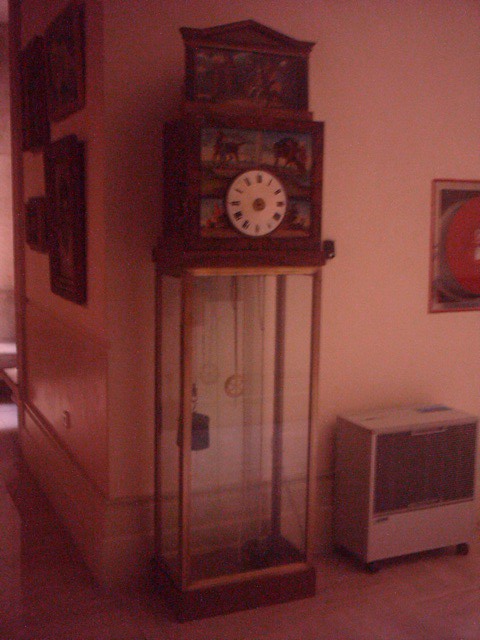This sepia-toned photograph, likely an old image with muted and almost reddish hues due to the incorrect white balance, showcases a portion of an open-plan living room or hallway. Dominating the scene is an extraordinary, African-themed grandfather clock. This ornate timepiece features a vividly detailed, temple-shaped top with colorful animal murals. The clock face, adorned with black Roman numerals set against a white background, is larger than typical grandfather clocks. Below the clock face, a glass display cabinet houses a small pendulum, adding to the clock’s distinct visual appeal with its brass-framed compartments. Surrounding the clock, a couple of indistinct pieces of wall art add subtle character to this cozy interior. Possibly an old-fashioned oil heater sits unobtrusively on the floor to the right, completing this nostalgic snapshot.